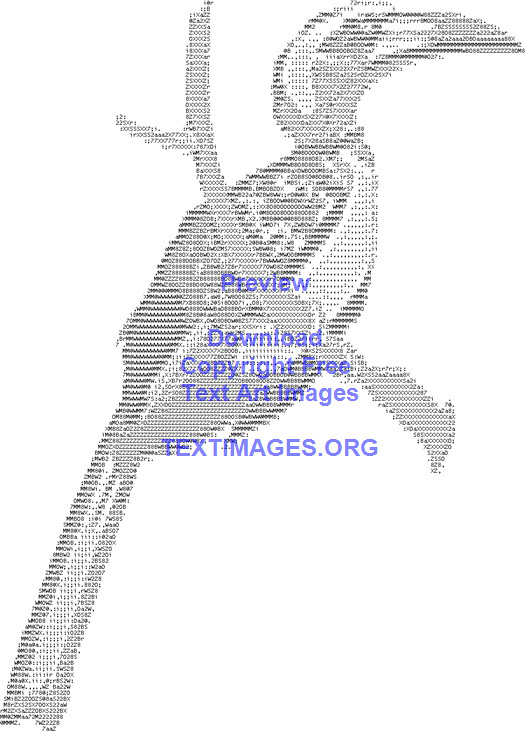The image features a black-and-white representation of a toucan perched on a branch, crafted entirely from various letters, numbers, and punctuation marks. Both the bird and the branch appear almost transparent, allowing the white background to show through their forms. The toucan is depicted with its characteristic long beak, a long tail, and contrasting black wings. The intricate text art gives the appearance of being computer-generated or pixelated. Above the bird in blue text, the words "preview, download, copyright free, text art images, textimages.org" are displayed, indicating that the image is available for use from the specified website. The toucan is shown looking to the right, with some foliage visible on the branch it’s perched on, giving a sense that it's either resting or ready to take flight.